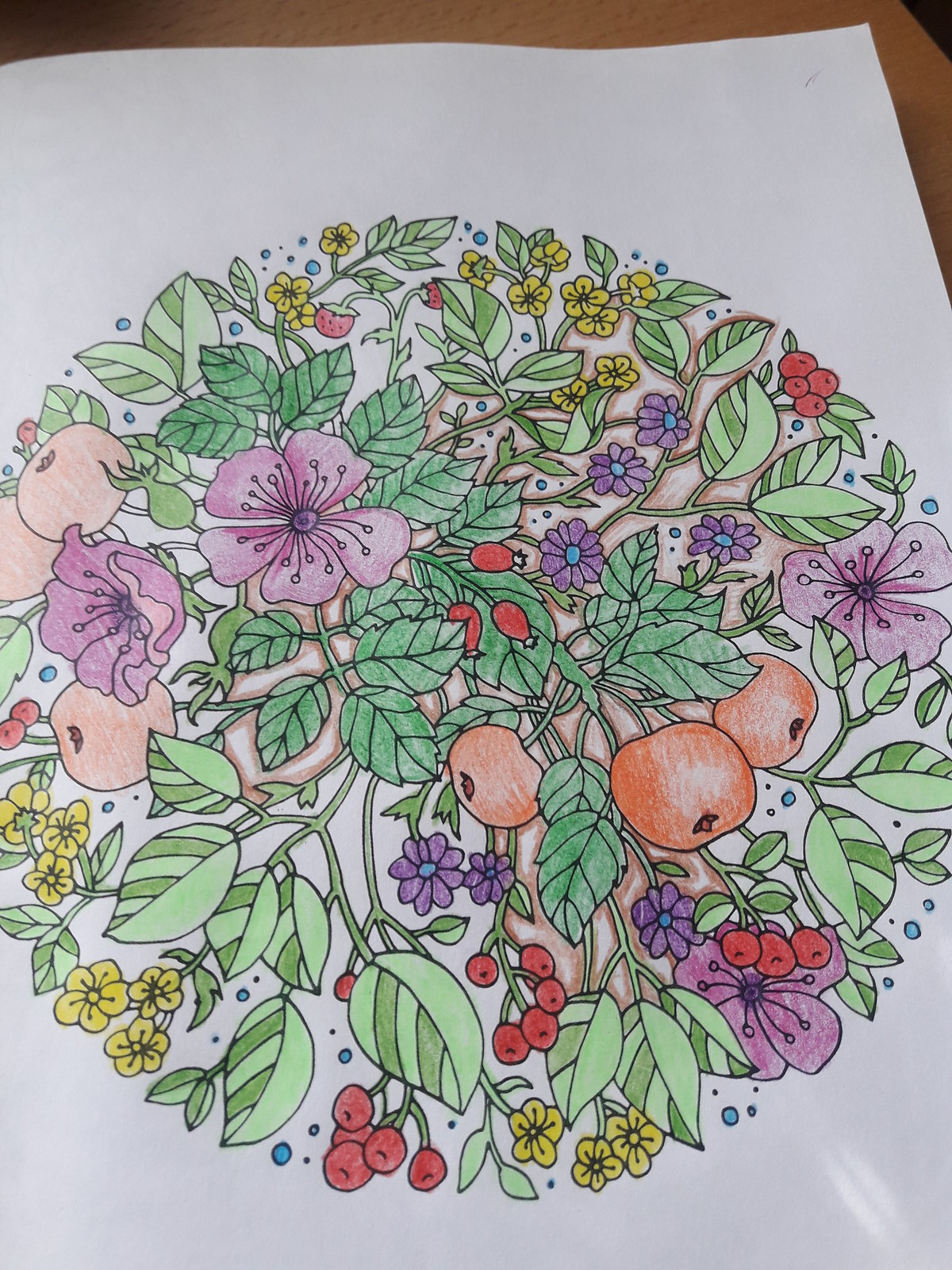This intricately designed illustration, resembling a page from an adult coloring book, features a circular composition filled with vibrant flowers, fruits, and leaves. The artwork, created on a clean white sheet of paper, is meticulously contained within a perfect round border, ensuring that no element extends beyond the edge. 

Within this harmonious circle, a variety of flora and fruit are showcased. Prominent among them are delicate pink hibiscus flowers, lending a tropical flair to the piece. Interspersed with these are fruits resembling apples or peaches, alongside clusters of red berries, possibly cherries, adding a burst of color and texture. 

Smaller yellow and purple flowers provide contrast and variety, while an abundance of lush green leaves fills the spaces between, contributing to the vibrant and cohesive appearance of the drawing. Certain areas of the illustration feature a subtle pink tint in the background, enhancing the depth and richness of the overall composition, despite the white paper base. This detailed and thoughtfully colored artwork captures the beauty and diversity of nature in a single, captivating round frame.